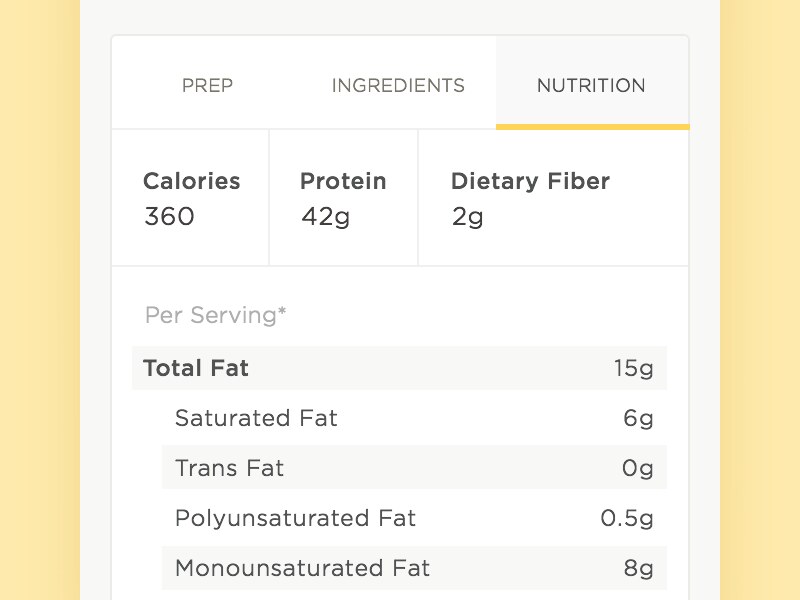The image depicts a detailed nutrition label with a structured layout. At the top, there is a gray square section titled "Prep and Ingredients." Beneath it, a yellow line demarcates the beginning of the nutritional information. The label is divided into three main columns: on the left, it displays "Calories," in the center, "Protein," and on the right, "Dietary Fiber."

- **Calories:** 360
- **Protein:** 42 grams
- **Dietary Fiber:** 52 grams

Below this section, the label mentions it's "per serving" in a star. There's a gray rectangle on the left labeled "Total Fat," with the following details:

- **Total Fat:** 50 grams
- **Unsaturated Fat:** 6 grams
- **Trans Fat:** 3 grams
- **Polyunsaturated Fat:** 0.5 grams
- **Monounsaturated Fat:** 8 grams

The label is bordered with a yellow strip on both left and right sides, and it has a tan coloring background. The inner section of the label maintains a light gray border surrounding the nutritional information, with a white background inside for clear readability.